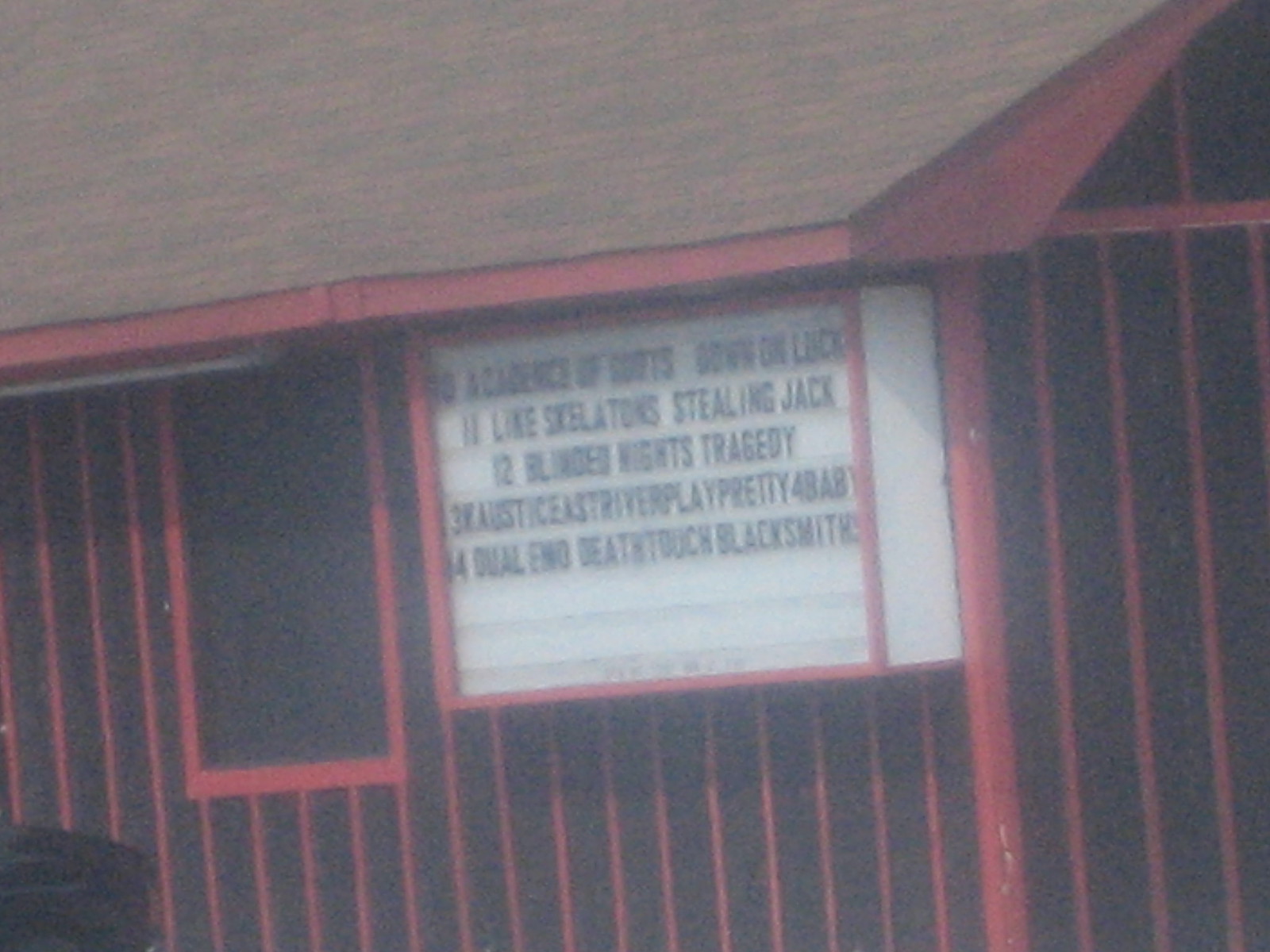The image depicts the exterior of a wooden building with a notably red and black security grill facade. The roof is covered in brown shingles, exhibiting hues of black and reddish-brown. Dominating the side of the building is a large, illuminated white sign framed in red, displaying black text, though its complete content is partially obscured and not entirely clear. The sign appears to list items or events in a random sequence, mentioning "number 11: skeleton stealing Jack," "number 12: blinded knights tragedy," "number 13: river play pretty baby," and "number 4: dual end death touch blacksmiths," potentially hinting at a list of movies. The photo quality is poor, with significant blurriness and a grayish haze, possibly due to smoke on the lens, making the details less discernible. A shadowy figure or a black shadow is visible in the bottom left corner of the image.